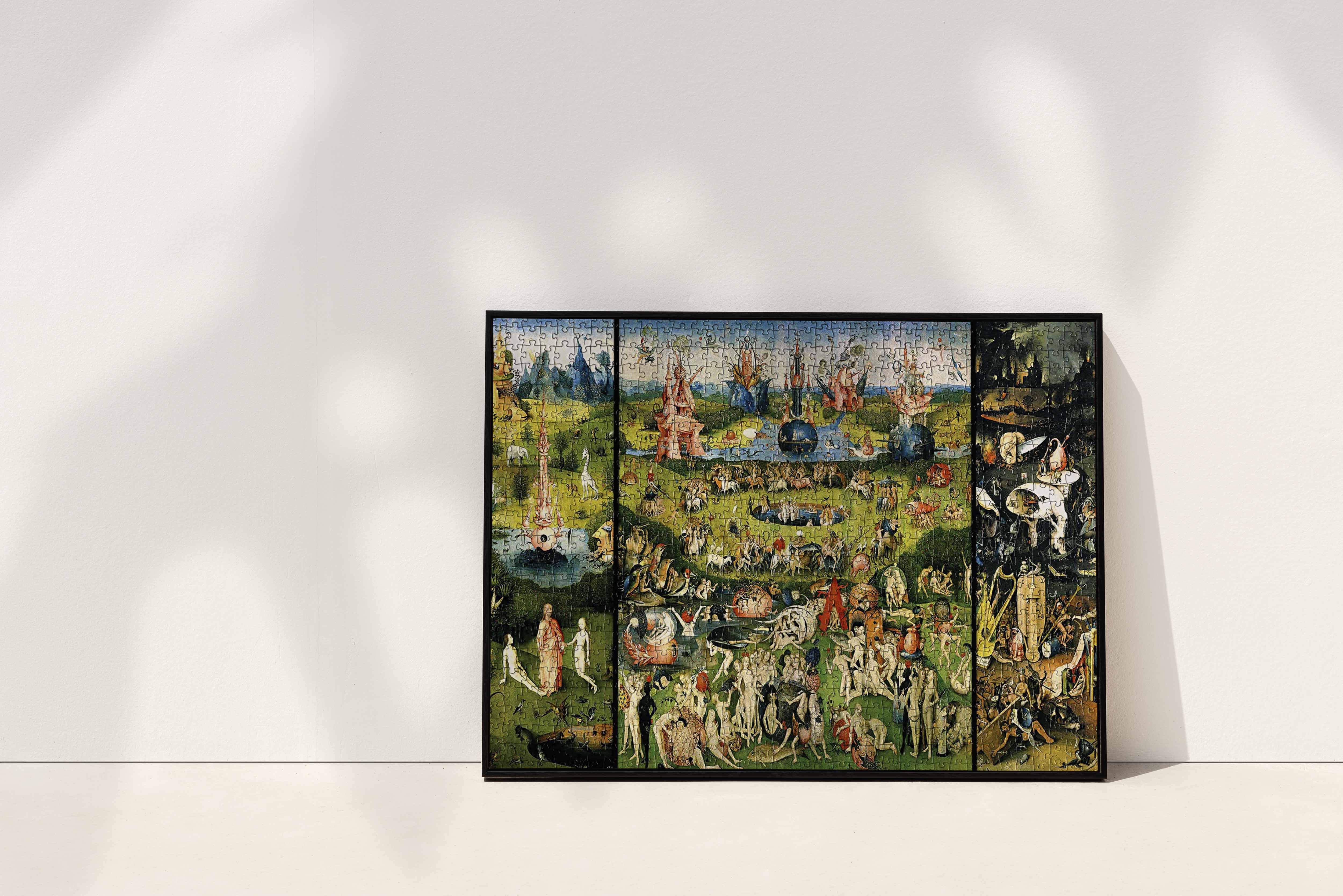The image depicts a meticulously assembled jigsaw puzzle of a famous triptych painting, possibly "The Garden of Earthly Delights" by Hieronymus Bosch, showcased in a black frame. The puzzle, carefully glued and framed, captures the intricate details of the early Victorian era artwork known for its surreal and obscure imagery. The scene is teeming with numerous naked figures engaged in various activities across a fantastical outdoor setting. On the left, three naked individuals conversing near a statue with a towering obelisk extending skyward can be seen. The central area features a group seemingly celebrating around a pool, surrounded by strange architectural structures and a lake. The right side portrays a chaotic scene with figures, potentially clothed, involved in what appears to be a battle or dance with sticks around a peculiar building. This complex tableau is set against a backdrop of sky and water, all grounded on a grassy expanse. The puzzle, leaning against a white wall and floor, casts subtle shadows, hinting at additional elements beyond its detailed imagery.